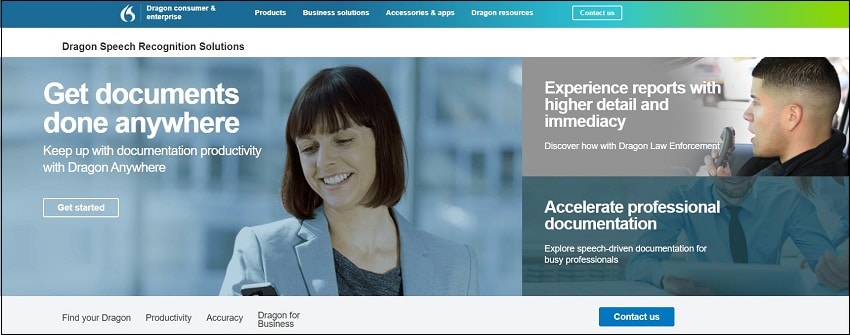In this captured image, we see what appears to be a screenshot from a computer screen showcasing various features and offerings of Dragon Speech Recognition Solutions.

At the very top of the image, there's a blue bar that transitions to green from left to right. Inside this bar, white text reads: "Dragon Consumer and Enterprise," "Products," "Business Solutions," "Accessories and Apps," "Dragon Resources," and a "Contact Us" button.

Below the blue bar, there's a white bar with black text that prominently states "Dragon Speech Recognition Solutions."

The main content is divided into three sections. The left section, occupying about two-thirds of the space, has a blue background with white text that reads: "Get Documents Done Anywhere. Keep up with documentation productivity with Dragon Anywhere." Below this, there is a "Get Started" button. The image in this section shows a woman looking down at a phone. She is dressed in a light powder blue blazer and a gray shirt, with chin-length brown hair and bangs. Only the top part of the phone is visible.

The right section is split into two smaller stacked boxes. The top box focuses on law enforcement and has white text on a darker background that says: "Experience Reports with Higher Detail and Immediacy. Discover How with Dragon Law Enforcement." The accompanying image features a man with a military-style shaved haircut, seemingly talking into a phone and looking to the left.

The bottom box in the right section promotes professional documentation, with white text on a dark background stating: "Accelerate Professional Documentation. Explore speech-driven documentation for busy professionals." The background image here shows a man in a suit, mostly focusing on his chest, arms, and chin.

At the very bottom of the image, additional text reads: "Find Your Dragon," "Productivity," "Accuracy," "Dragon for Business," and there is a blue "Contact Us" button.